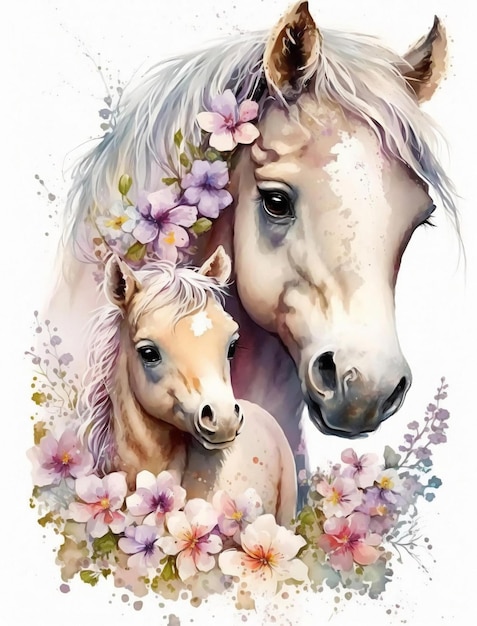A beautifully rendered illustration captures the gentle bond between an adult horse and its foal. The artwork, which exhibits a delicate watercolour style, might be either digitally generated or meticulously hand-painted. The colour palette consists of muted, pastel hues that evoke a sense of calm and tranquility. The two horses, one mature and the other a young foal, stand intimately close, with the foal positioned protectively under the adult horse. Both animals possess long, wispy white manes that cascade gracefully, and their coats are subdued shades of light brown and grey, blending seamlessly with the ethereal background. Encircling the serene equine pair are an array of vividly coloured flowers, predominantly in soft purples and pinks, which add a floral elegance and vibrancy to the composition. The overall effect is a harmonious and tender scene that captures the beauty of nature and the gentle relationship between the horses.